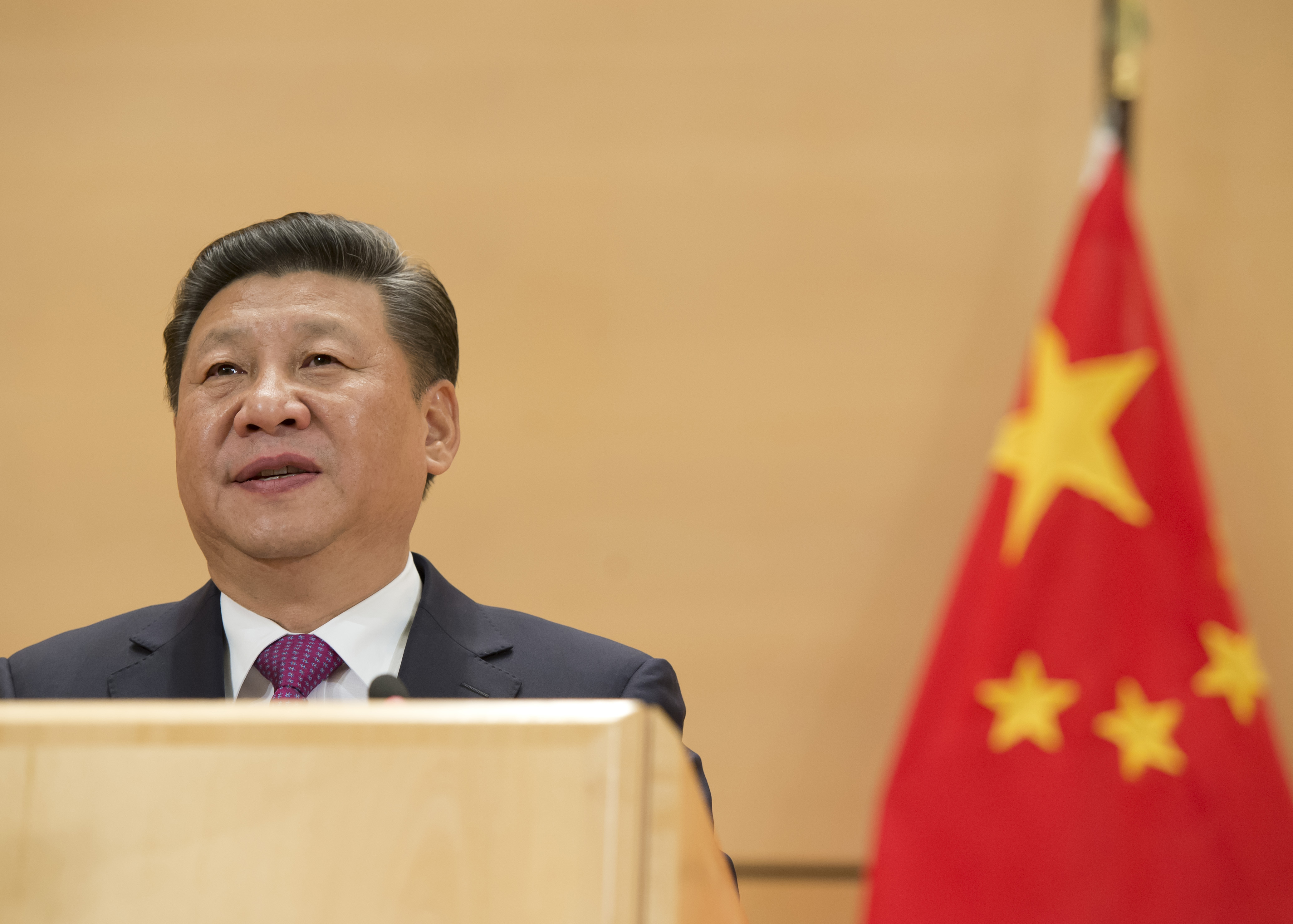A man of Asian descent stands assertively behind a beige podium that blends seamlessly with the similarly colored background wall. He has a neatly trimmed, short haircut that complements his round face and large neck. His chin subtly merges into his neck, giving him a distinguished look. He is impeccably dressed in a black suit jacket over a crisp white button-up shirt, accentuated by a purple tie adorned with polka dots. Just beside him, a flag on a flagpole displays a striking red background with one prominent yellow star at its center and three smaller yellow stars below it, adding a vibrant splash of color to the scene.